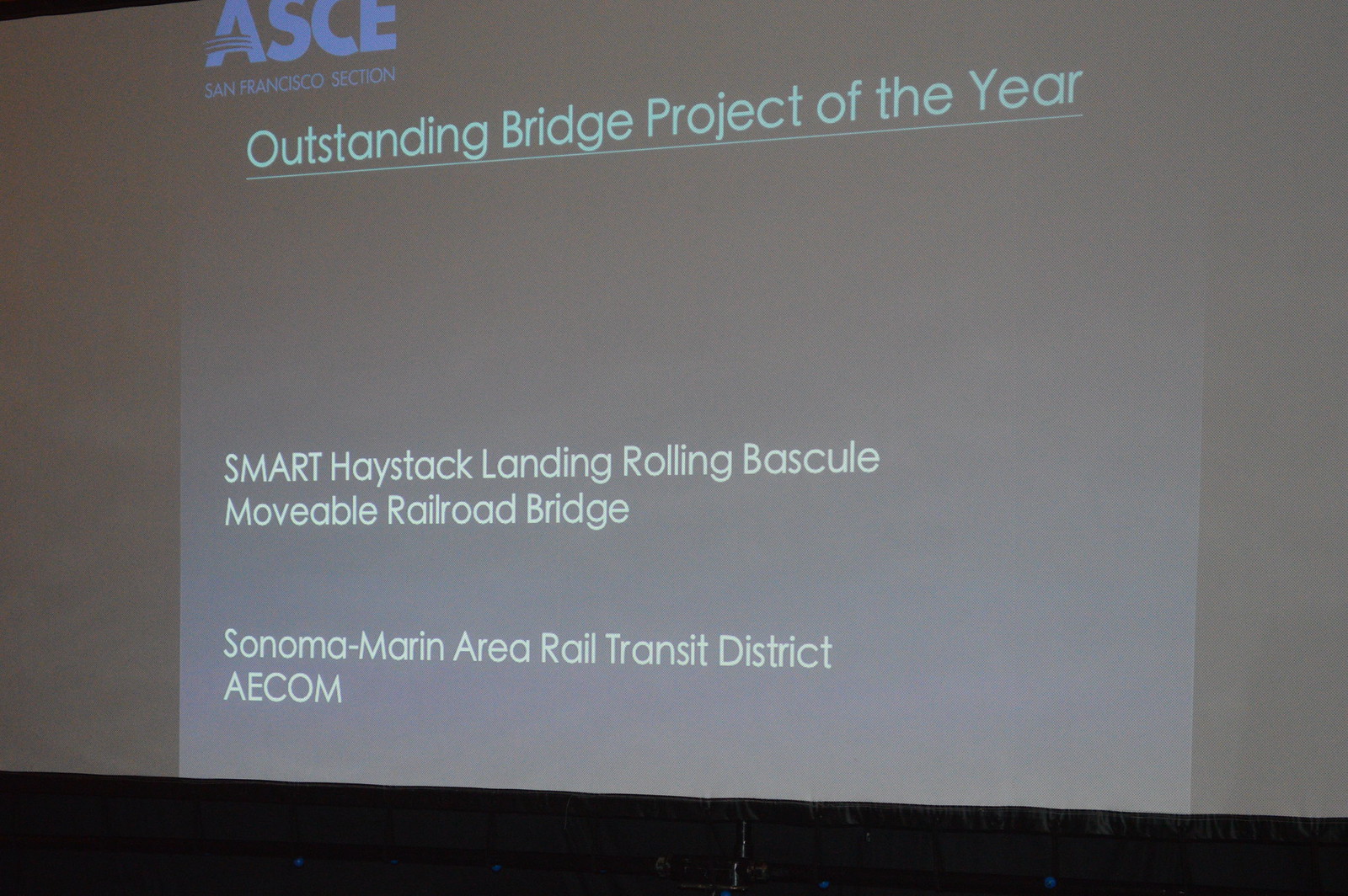The image features a projected presentation slide with a predominantly dark background. In the top left corner, the blue brand logo "ASCE" is displayed, with the "A" stylized with three lines extending left and right below its center. Below the logo, it reads "San Francisco Section." The title of the slideshow is prominently placed in the middle of the screen, underlined, and says "Outstanding Bridge Project of the Year" in light green text. Central to the slide, in off-white lettering, it states "SMART Haystack Landing Rolling Bascule Movable Railroad Bridge." Further down, the slide identifies "Sonoma-Marin Area Rail Transit District," followed by "AECOM" in all caps. The left, right, and background areas of the slide are primarily black, giving the main content a striking contrast against its gray backdrop.